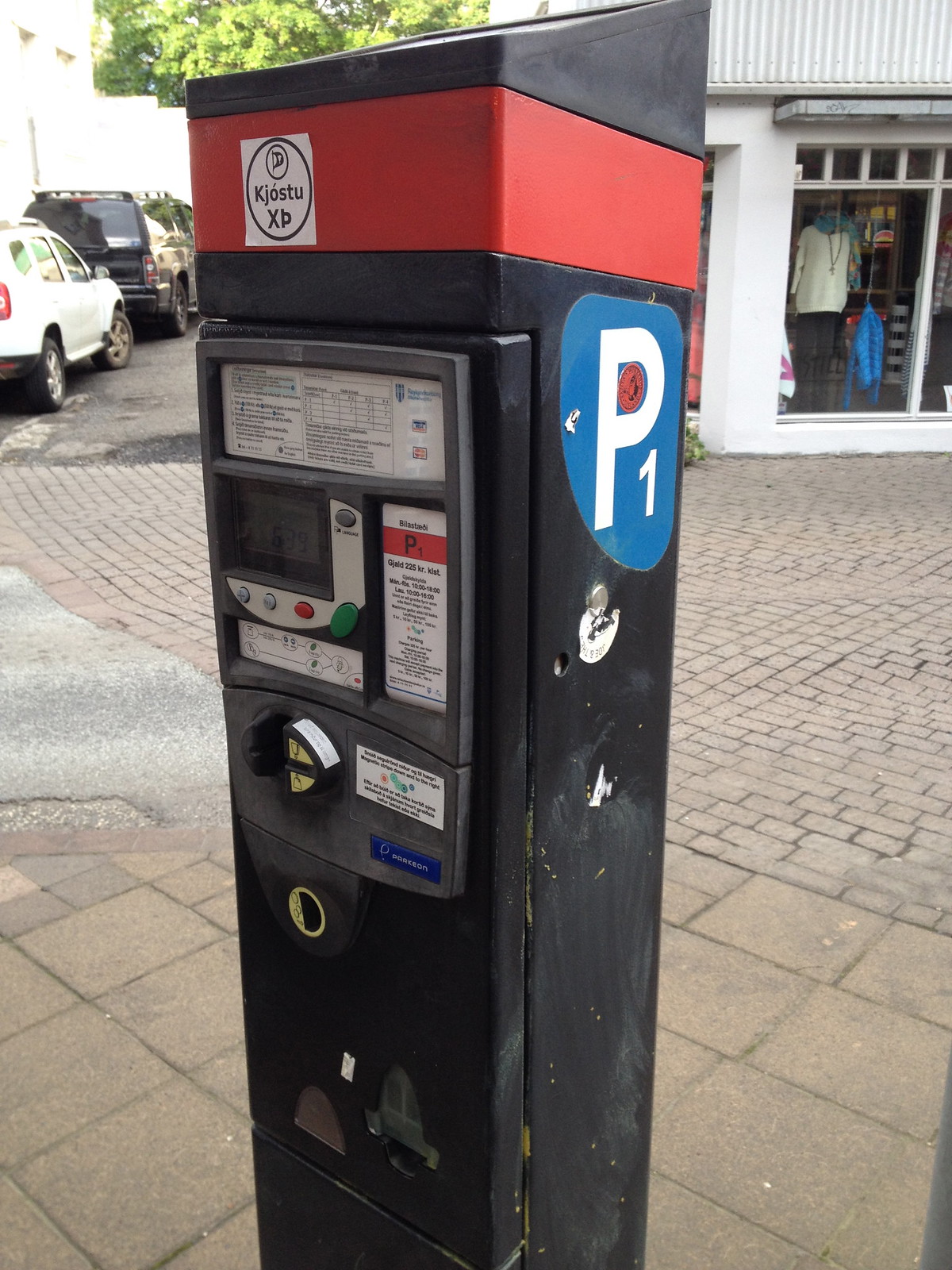This vibrant outdoor photograph captures a bustling shopping district, where a prominent parking ticket dispenser stands as the focal point on a cobblestone sidewalk. The dispenser is black with a distinctive red stripe at the top and features a blue circular sticker bearing a white "P1" on its side. The device's front panel includes a digital LED display and a slot for credit and payment cards, accompanied by instructions in white text. In the background, a large store is visible through its full glass window, showcasing a mannequin dressed in black pants, a cream-colored shirt, and a blue and yellow scarf, accessorized with a long necklace with a cross. A blue puffer jacket hangs next to the mannequin. To the left, a line of parked cars is seen, with a lush, leafy tree adding a natural element to the urban scene.